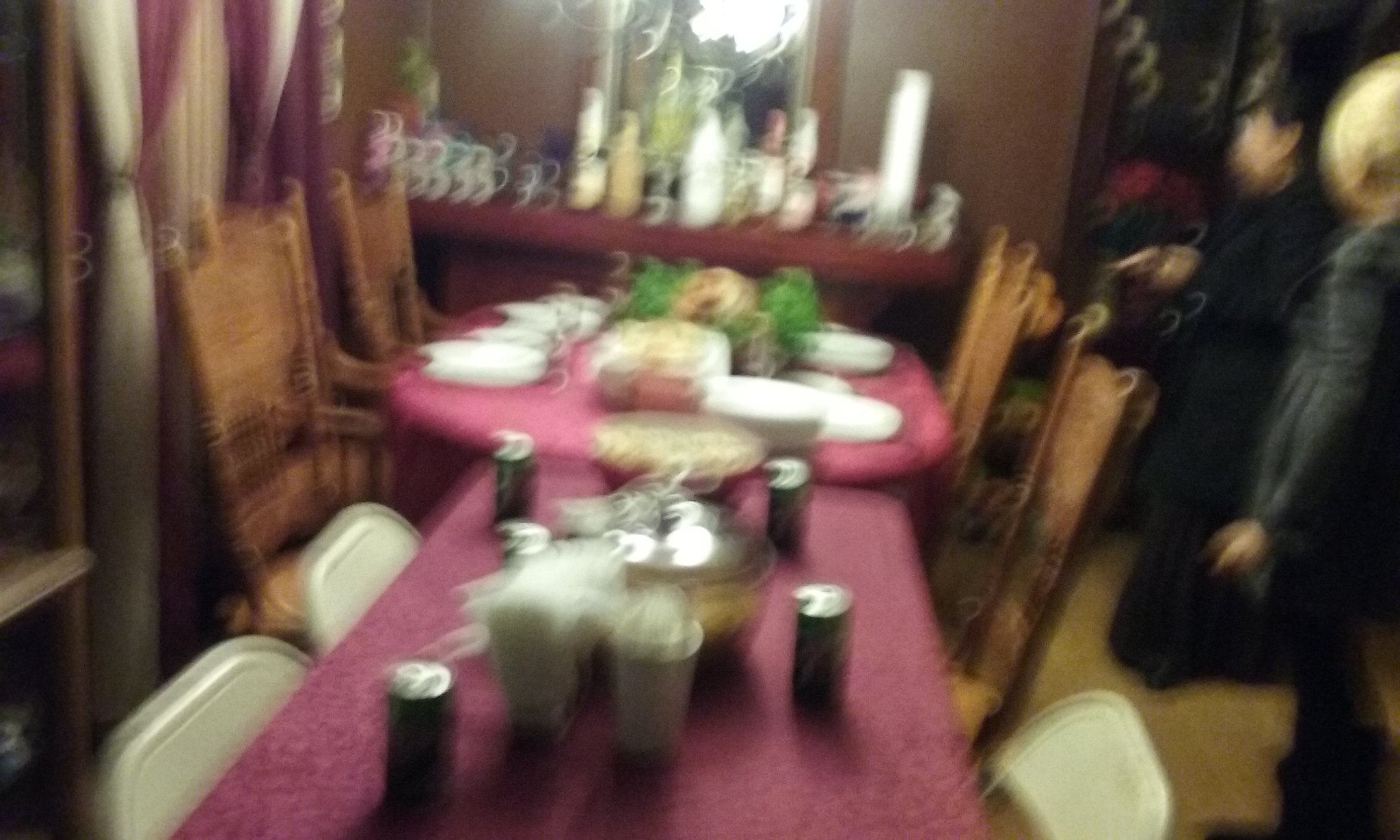This image is a blurry photograph of a small, well-lit dining room, probably in a home. The focal point of the image is a dining arrangement made up of two tables pushed together. One table is a long rectangular shape situated closest to the bottom of the photograph, and the other is a slightly wider, rounded table. Both tables are draped with burgundy-colored tablecloths.

The rectangular table has three folding metal chairs in a beige color, while the rounded table is surrounded by four high-backed wooden chairs. On the rectangular table, there are four cola cans and some plastic cups that might be holding napkins, along with a couple of large bowls similar to those found at a potluck. The rounded table features place settings with white plates, glasses, and some greenery as a centerpiece.

In the background, there is a smaller table against the wall, possibly a buffet table or a bar area, on which several stacks of white cups and other items are placed. This table is topped by a mirror. To the left of the image, maroon and white curtains adorn the window, and on the right-hand side, two people, one in a long gray dress and the other in a long black dress, are standing, perhaps waiting to be seated. Behind them, there appears to be a brown door and another piece of furniture, possibly a shelf.